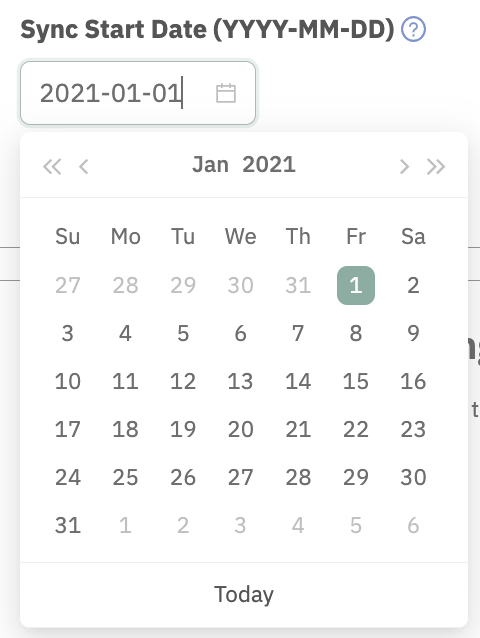The image captures a detailed close-up of a calendar pop-up interface within an application. The photo, taken in portrait orientation, lacks defined borders or a background, focusing solely on the calendar pop-up element. 

At the top of the interface, the text "Start Sync Date" is displayed in black font, followed by the date format "YYYY-MM-DD" in parentheses. Adjacent to this text is a blue circle containing a white question mark, serving as a help icon. Below this, there is a date input field, outlined with a green border and featuring a rectangular shape with rounded corners. The selected date is "2021-01-01."

A calendar pop-up enables users to conveniently scroll and select a date rather than manually typing it in. In this instance, the month displayed is January 2021. Navigation arrows on either side of the month allow the user to switch between different months and years – double arrows likely shift the view by a year, while single arrows adjust it by a month. Below the calendar interface, the word "Today" indicates the current date, which corresponds to January 1, 2021.

Within the calendar, the days of January are clearly visible against a white background. Days from other months appear grayed out. The selected date, January 1st, is highlighted with a green box featuring rounded edges and a white number inside, indicating it is the chosen date within the interface.